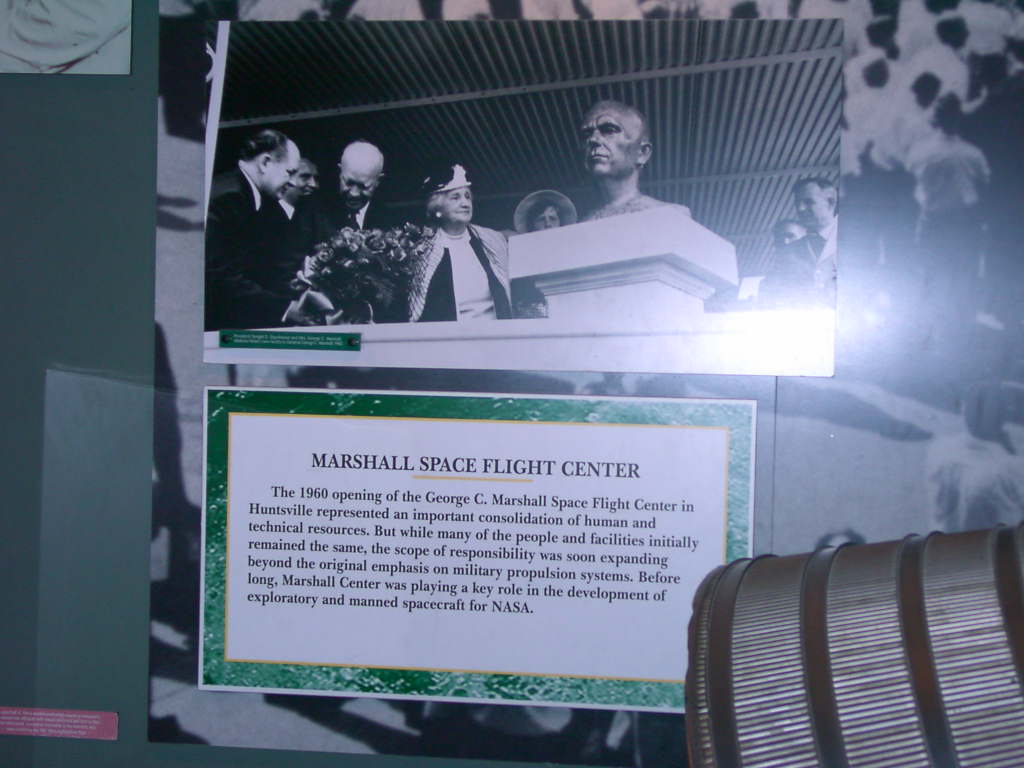The image depicts a black-and-white photograph featuring multiple people observing a bust statue of a man, with some individuals holding floral arrangements. The attire of the people suggests that the photograph is from an older era. Behind the bust, more individuals can be seen, all contributing to the scene's historical atmosphere. The backdrop appears to include some metal elements. Below the photograph, an informational placard reads: "Marshall Space Flight Center. The 1960 opening of the George C. Marshall Space Flight Center in Huntsville represented an important consolidation of human and technical resources. While many of the people and facilities initially remained the same, the scope of responsibility was soon expanding beyond the original emphasis on military propulsion systems. Before long, Marshall Center was playing a key role in the development of exploratory and manned spacecraft for NASA." The sign is in black, white, yellow, and green colors, providing contextual details about the significance of the Marshall Space Flight Center.